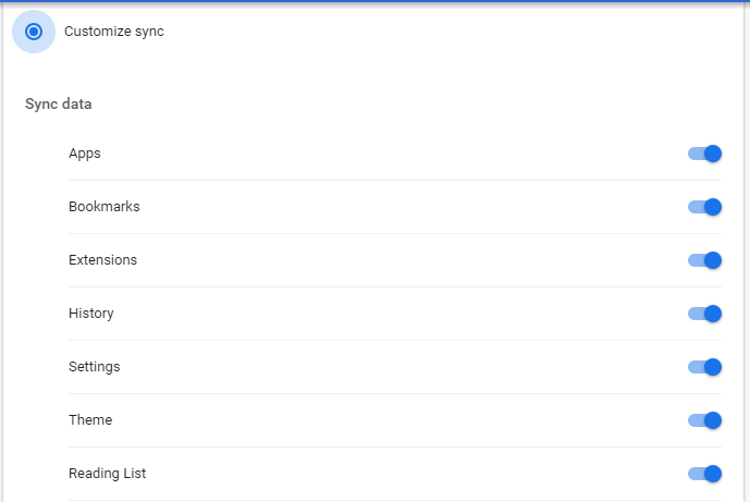Screenshot of a sync customization page, likely from a settings menu within an unknown app or browser. The page has a clean white background, featuring a title "Customize Sync" highlighted with a blue dot and adjacent black text at the top. Below the title, the section is labeled "Sync Data," which lists seven distinct data categories: Apps, Bookmarks, Extensions, History, Settings, Theme, and Reading List. Each category is equipped with a toggle switch on the right, all of which are currently turned on and highlighted in blue, indicating that all sync options are activated.